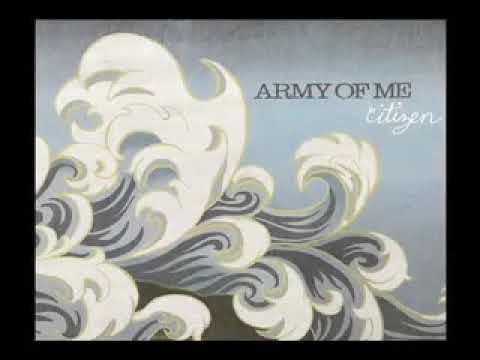This album artwork for the band Army of Me features a striking illustration of crashing ocean waves. The waves, which are predominantly white with dark navy blue swirls and hints of gray and beige, appear almost animated and painted with an artistic touch. They dominate the canvas, sweeping up to the top and curling down towards the right, bordered by a deep black frame. The background is a cloudy gray, enhancing the dynamic and turbulent feel of the waves. At the top, in bold capitalized letters, "ARMY OF ME" is prominently displayed in gray. Beneath this, in a cursive, handwritten white script, is the word "Citizen," adding a delicate contrast to the boldness above. The overall composition is evocative, blending the raw power of nature with the finesse of artistic expression, making for an intriguing album cover.